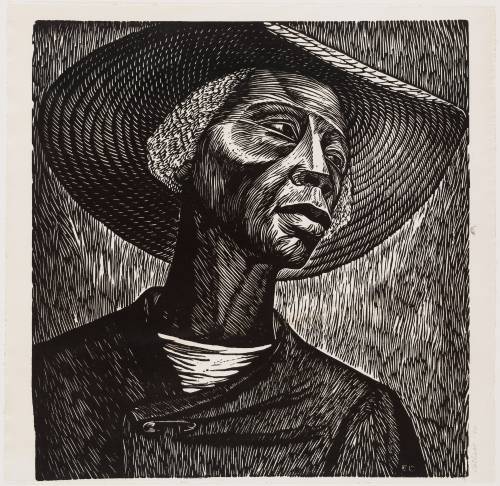The artwork is a detailed black and white etched portrait, likely of a black person, possibly an older African-American woman. The individual is wearing a large, floppy sun hat that suggests an outdoor setting, possibly a utilitarian accessory for a peasant or worker to shield against the sun. The portrait employs intricate crosshatching techniques, creating rich gradations of black, white, and gray. It appears to be an older style, reminiscent of art from over a century ago. The figure, with a broad nose, full lips, and a graceful, long neck, gazes into the distance with a somber expression. She wears a coat secured with a safety pin over what looks like a white t-shirt. The background is composed of various shades, enhancing the depth and texture of the image. The overall impression is of a dignified yet weary figure, capturing a moment of still contemplation.